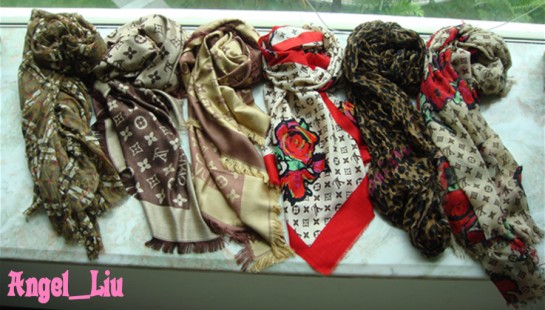The photograph features an artfully arranged collection of seven scarves laid out on a white scarf adorned with gray squares, crosses, and diamond shapes, set against a gray cement background. Extending across the center of the white scarf from left to right are six additional scarves, each varying in color and pattern: starting with a greenish-gray scarf, followed by a dark brown and tan one, then a beige scarf with brown and creamy yellow accents. At the center lies a white scarf bordered in red, featuring what looks like lips and a rose petal print. To its right is a ruffled scarf with a cheetah print, and on the far right, a tan-colored scarf with intricate darker gray-brown patterns and red accents. The display sits atop a greenish-hued surface, and in the bottom left corner, "Angel_UnderScore_Loo," spelled L-O-O-O, is prominently written in pink letters.